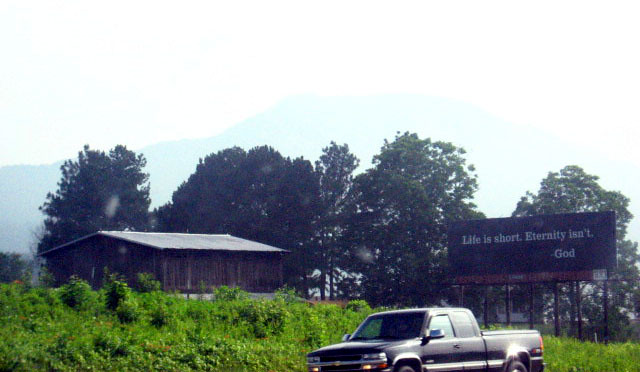In this detailed photograph of a rural landscape, a black truck can be seen driving along a country road. The truck's presence is contrasted by the lush green hill beside it, which is covered in dense vines, likely kudzu. Nestled beyond this verdant hill is a quaint, rustic wooden house that exudes a sense of simplicity and tranquility. A row of trees stands tall behind the house, providing a natural backdrop that enhances the pastoral scenery. In the distance, the horizon is adorned with a mist-shrouded mountain, adding a touch of mystique to the landscape. Adjacent to the house is a prominent billboard bearing the message: "Life is short. Eternity isn't. God," in a bold, reflective statement that invites contemplation against the serene setting.